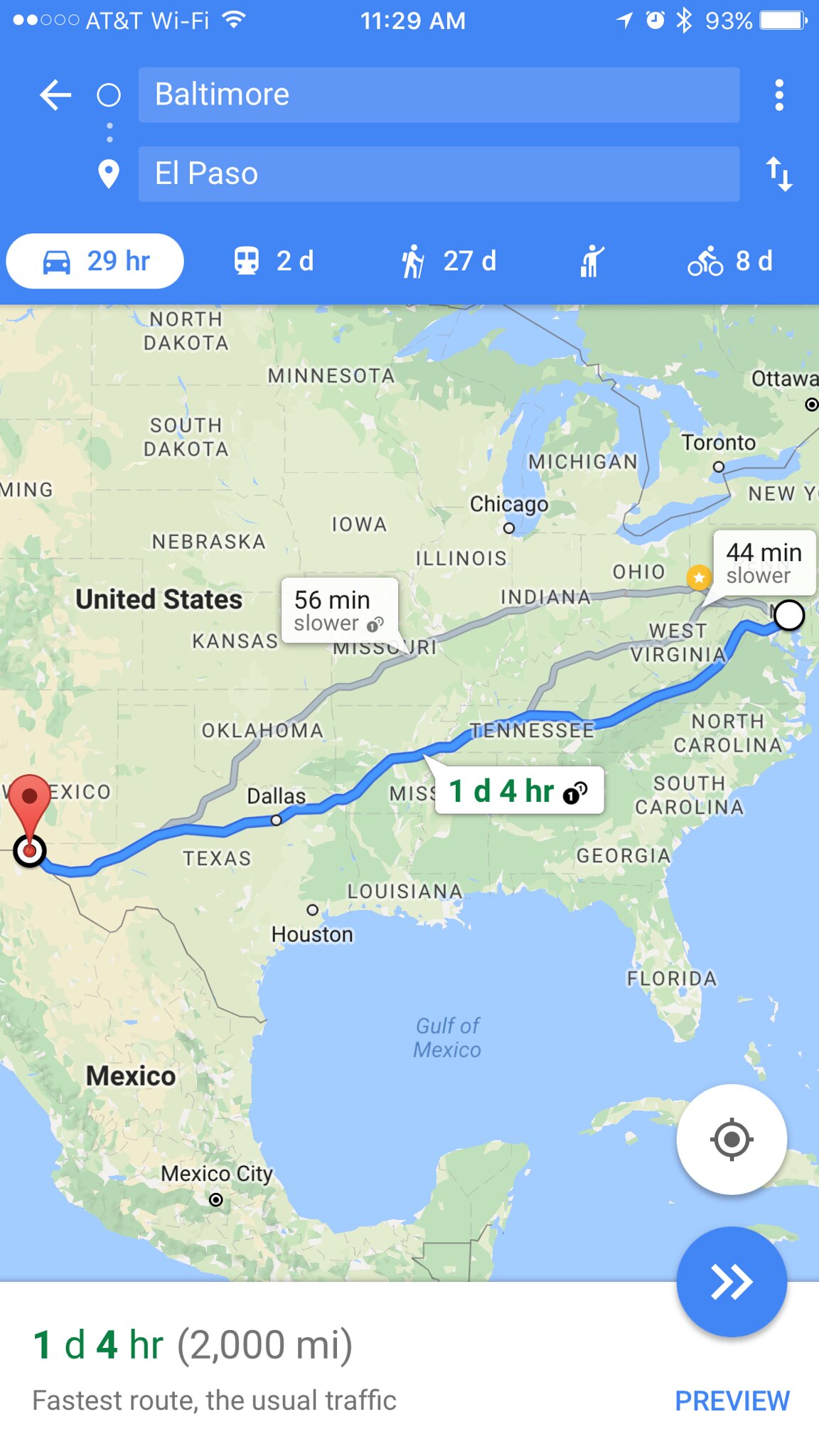The image displays a smartphone screen featuring a navigational map, likely from Google Maps or MapQuest, plotting a route from Baltimore, Maryland to El Paso, Texas. The prominent blue line delineates the travel path across several states. The screen indicates the total travel time as one day and four hours, while a white button in the corner, accompanied by a car icon, shows an alternative duration of 29 hours. The map spans a significant portion of the United States, including visible portions of the Gulf of Mexico and the Atlantic Ocean. Additional details at the top of the screen reveal the user is connected to AT&T Wi-Fi, with the current time being 11:29 a.m., and the device's battery is at 93%.